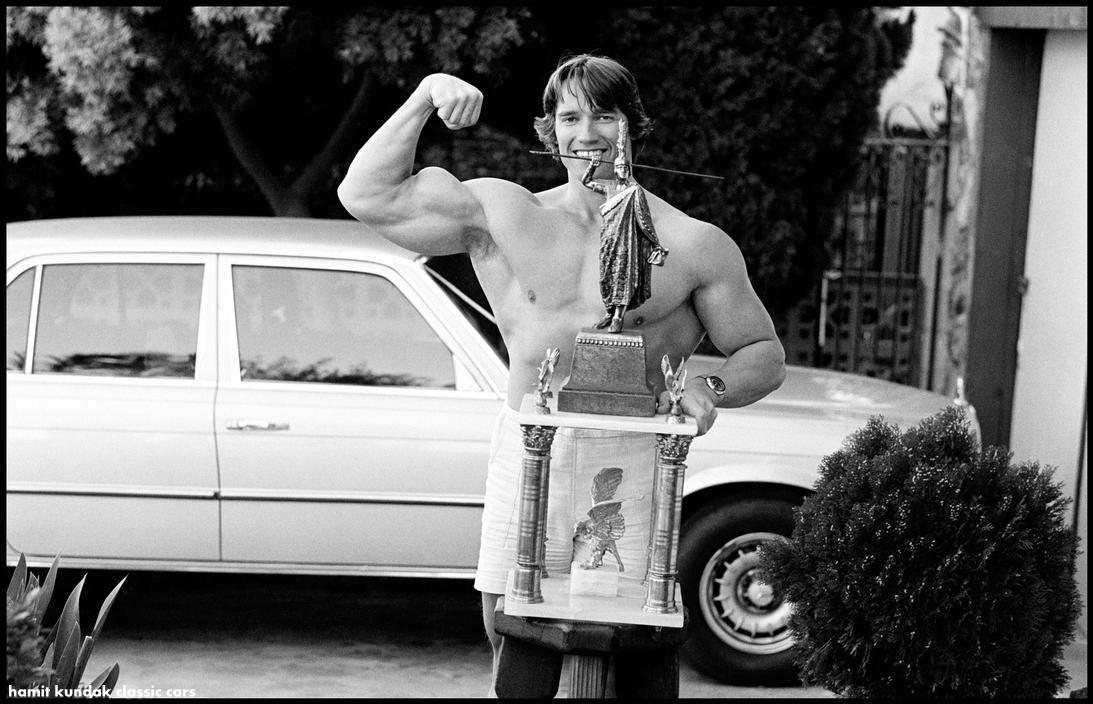This black and white photograph, likely from the 1970s or 80s, captures a young and physically fit Arnold Schwarzenegger standing proudly in front of a light-colored, boxy car parked in a driveway, with a garage and trees in the background. Arnold is shirtless, showcasing his impressive, well-built physique. He is prominently positioned at the center of the image, visible from his knees up. His right arm is flexed in a classic bicep pose, emphasizing his muscular build.

In his left hand, Arnold holds a towering trophy, approximately three feet tall, featuring intricate details. The trophy includes an eagle at the bottom, supported by pillars, and is crowned by a man in a toga and helmet, wielding a long spear or sword behind his head. The trophy's base appears to be resting on a pillar in front of Arnold. Additionally, Arnold is wearing a watch on his left wrist. The car, which might be a Mercedes, is oriented towards the three o'clock position, alongside some shrubbery. The entire scene is nostalgic, evoking a sense of Arnold’s early bodybuilding triumphs.